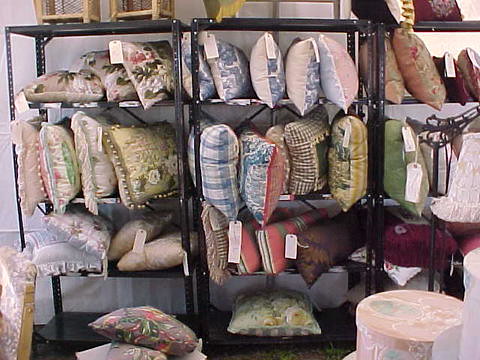The image depicts three dark gray metal shelving units, each with five shelves, standing against a light-colored wall. The shelves are laden with an assortment of decorative pillows, arranged neatly in varying numbers. The leftmost unit features three pillows on the top shelf, followed by four pillows on each of the next three shelves, with the bottom shelf empty. The middle unit holds five pillows on both its top and second shelves, four pillows on the third shelf, and a single pillow on the bottom shelf. The rightmost unit is partially visible, showing three pillows on the top shelf, one pillow on the second and third shelves, with the lower shelves obscured from view. The pillows come in a variety of colors including oatmeal, grays, blue checkered patterns, and floral designs. Some pillows have visible tags, and there's a prominent large red pillow at the bottom right corner. The shelving units contrast with a black floor and a white wall, creating a stark backdrop for the colorful pillows.